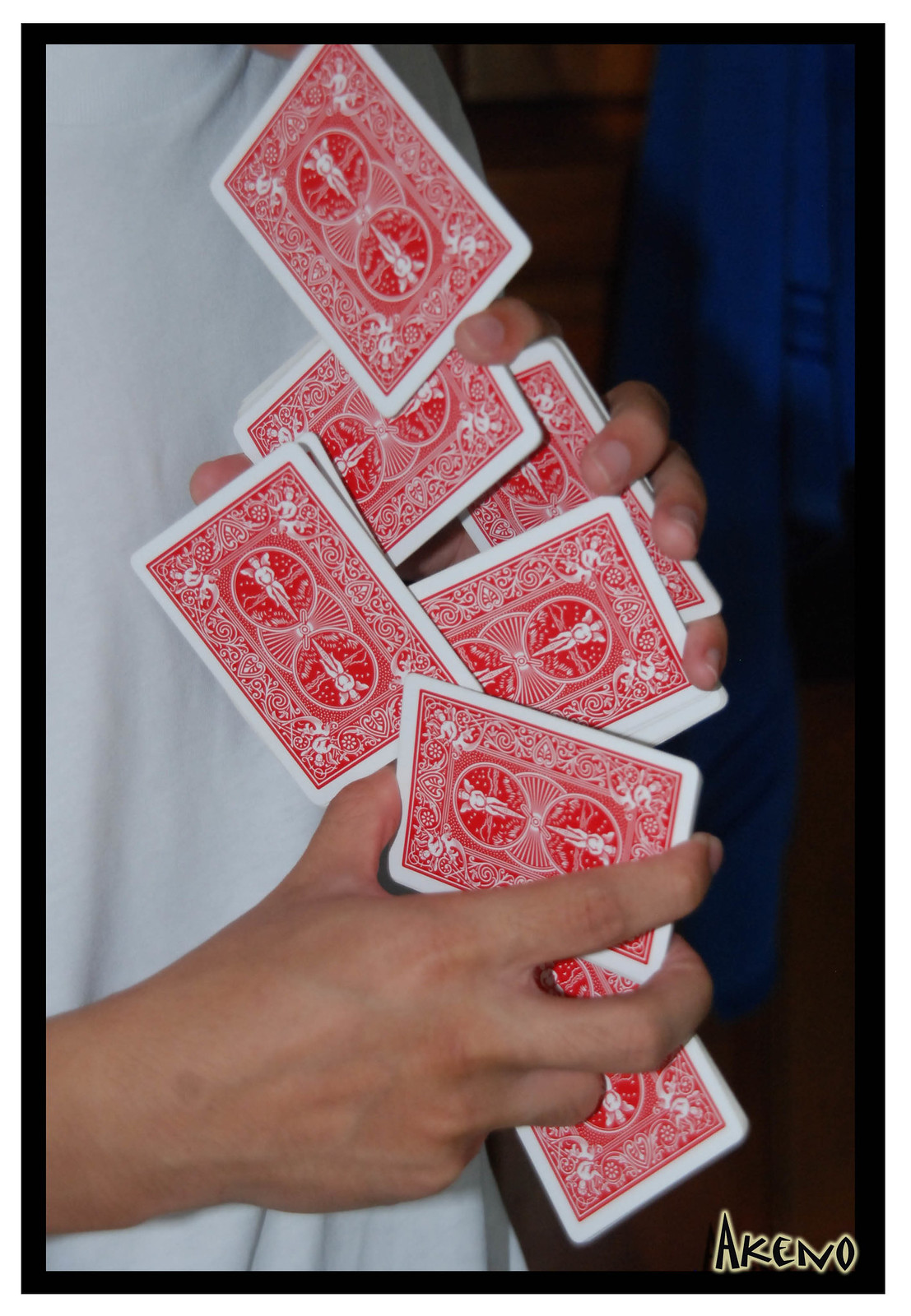A mesmerizing photograph captures a skilled magician mid-performance, executing an impressive card trick with exceptional precision. The image, framed by a sleek black border, features a striking black tag at the bottom that reads "Akino" in a tribal-style font, highlighted by a glowing yellow aura.

In the center of the frame stands the magician, a man of fair or tan complexion, effortlessly holding seven separate stacks of red Bicycle brand playing cards. Each stack is meticulously positioned at varying angles, showcasing his adeptness in handling the cards. Dressed in a crisp white shirt, the magician commands attention as he displays the familiar red backs of the playing cards, adorned with intricate designs featuring two angels, circles, and elaborate ornate details.

Standing beside him, an individual in a blue coat or shirt observes the captivating performance. The photograph, devoid of any motion blur, captures the moment in perfect clarity, emphasizing the magician’s remarkable steadiness and control. Although the suits and numbers remain hidden, the classic red Bicycle design on the cards adds a touch of nostalgia and authenticity to this enchanting scene.